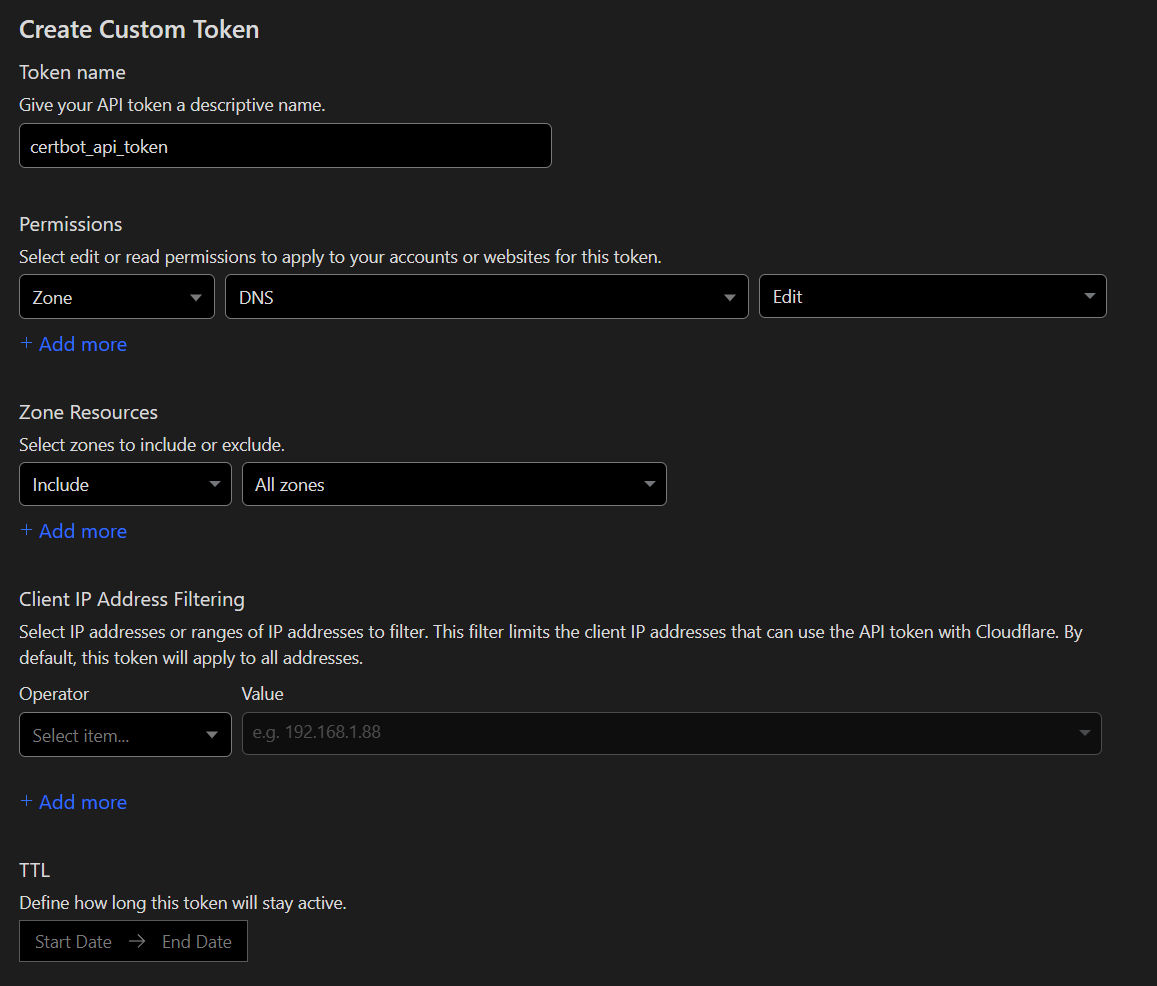This image depicts a control panel for creating a custom API token within the CloudFlare platform. The medium gray panel, accentuated with black input fields surrounded by light gray lines and featuring curved corners, is designed for user-friendly interaction.

At the top, users are prompted to provide a descriptive name for the API token, such as "certbot_API_token". Below this, in the permissions section, users can select from drop-down options to designate the token's permissions, such as "editor" and "read" permissions for accounts or websites, focusing specifically on "zone" and "DNS" with the ability to edit. Users can add additional permissions by clicking on the blue "Add more" text.

The next section, "Zone Resources," allows users to include or exclude specific zones. These zones can be selected from drop-down options with additional zones being added via another "Add more" feature.

Following this, there's the "Client IP Address Filtering" section. This feature enables the restriction of API token usage to specific IP addresses or ranges, with an example format of "192.168.1.88" provided in gray text. By default, the token applies to all addresses unless specified otherwise. Additional IP filters can be added using the "Add more" option.

Finally, users can define the token’s Time To Live (TTL), which determines how long the token remains active, specifying both the start and end dates in black input fields.

This comprehensive control panel by CloudFlare ensures robust security and precise management of API tokens.